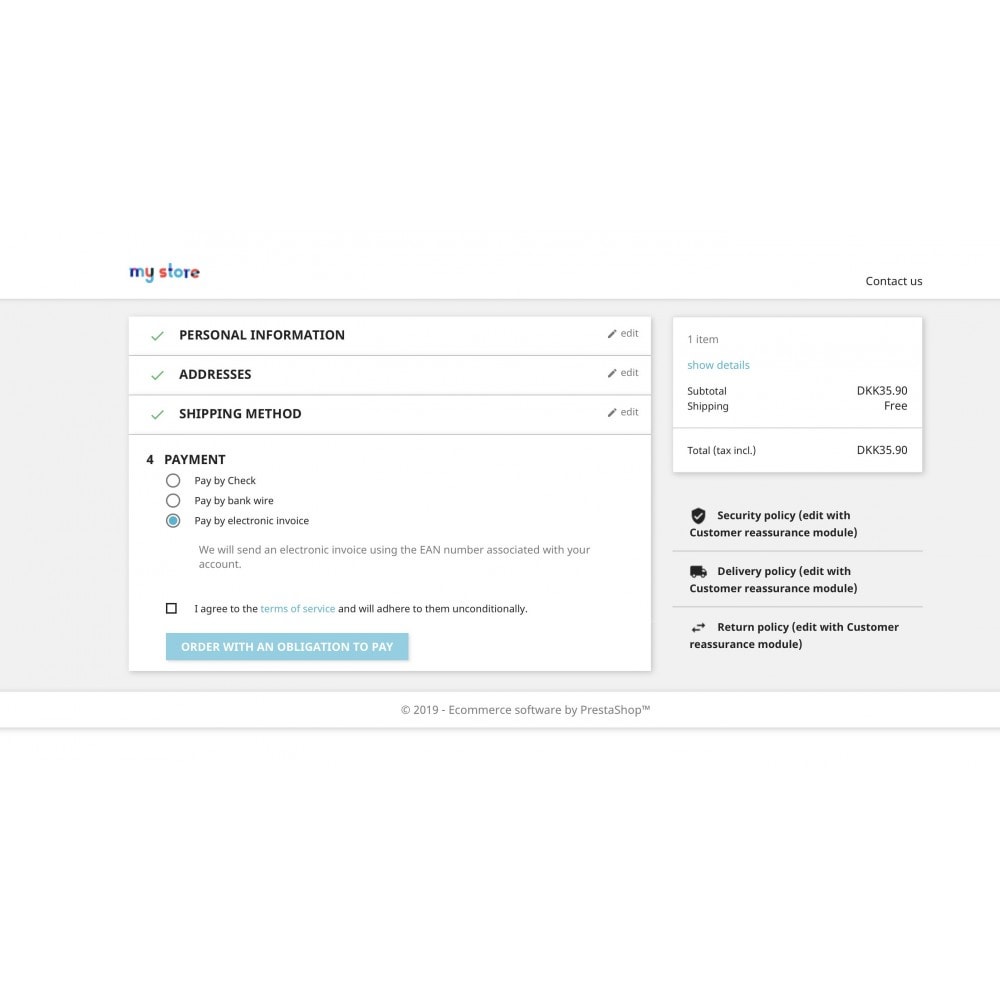This image appears to be a screenshot of an e-commerce checkout page from someone's computer. At the top of the screen, there's a large white banner. In the left corner of this banner, the colorful phrase "My Store" is displayed. The lettering is uniquely colored: the M is blue, the Y is a mix of red and blue, the S is red, the T and O are light blue, the R is dark blue, and the E is gray outlined in red. On the far right of the banner, there is a "Contact Us" link.

Below the banner, the screen is divided into two main sections within a gray rectangle. The left section features a series of steps in a white rectangle: at the top, "Personal Information" is listed with a checkmark to its left, followed by "Addresses" with a checkmark, then "Shipping Method" with a checkmark. Finally, the current step, "Payment," is highlighted as the fourth step. Under Payment, there are three options available: "Pay by Check," "Pay by Bank Wire," and "Pay by Electronic Invoice," with the latter option selected as indicated by a filled circle.

At the bottom of this left section, a blue rectangle button is labeled "Order with an Obligation to Pay."

The right section contains a white box displaying a summary of the order: one item with a subtotal of DKK35.90, free shipping, and a total amount of DKK35.90. Beneath the order summary, there are sections outlining the store's Security Policy, Delivery Policy, and Return Policy.